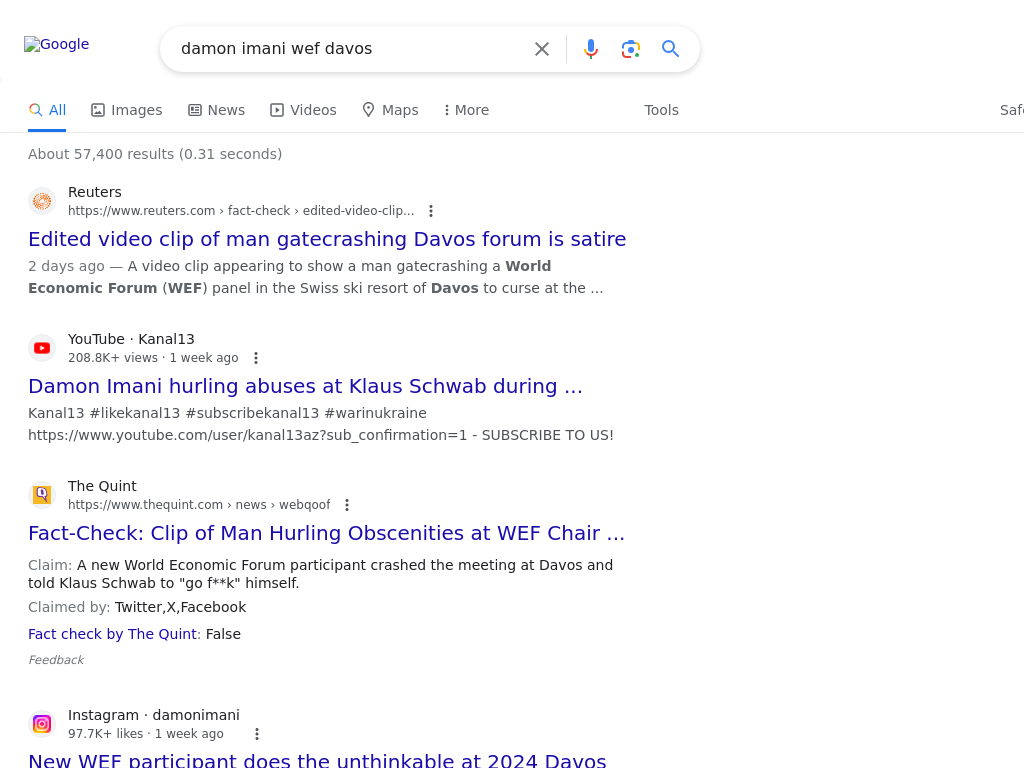This image is a screenshot of a computer screen displaying a Google search results page. In the top left corner, the "Google" logo is prominently visible. Centrally focused on the page is the search bar, which includes a small 'X' icon on the right end to clear the search query. Adjacent to the 'X' are three further icons: a microphone for voice search, a camera for image search, and the traditional magnifying glass search icon.

Below the search bar is a navigation menu with various tabs enabling different types of search results: "All," "Images," "News," "Videos," "Maps," "More," and "Tools." To the far right of this menu, only the left half of the word "Safety" is visible.

The search results indicate "About 57,400 results" in bold text, followed by the search duration in parentheses, "(0.31 seconds)." There are four visible search results on the screen:

1. The top result is from Reuters, featuring the headline "Edited video clip of man gate-crashing Davos Forum is satire," which is a clickable hyperlink. A brief description follows this headline.
2. The second result is a YouTube link titled "Damon Imani hurling abuses at Klaus Schwab during," also a clickable blue hyperlink.
3. The third result is from The Quint with the headline "Fact check: clip of man hurling obscenities at WEF chair," similarly formatted as a clickable hyperlink.
4. The fourth result, partially cut off at the bottom of the screen, is from Instagram. The visible part of the headline reads "New WEF participant does the unthinkable at 2024 Davos," but the description is not visible due to the cutoff.